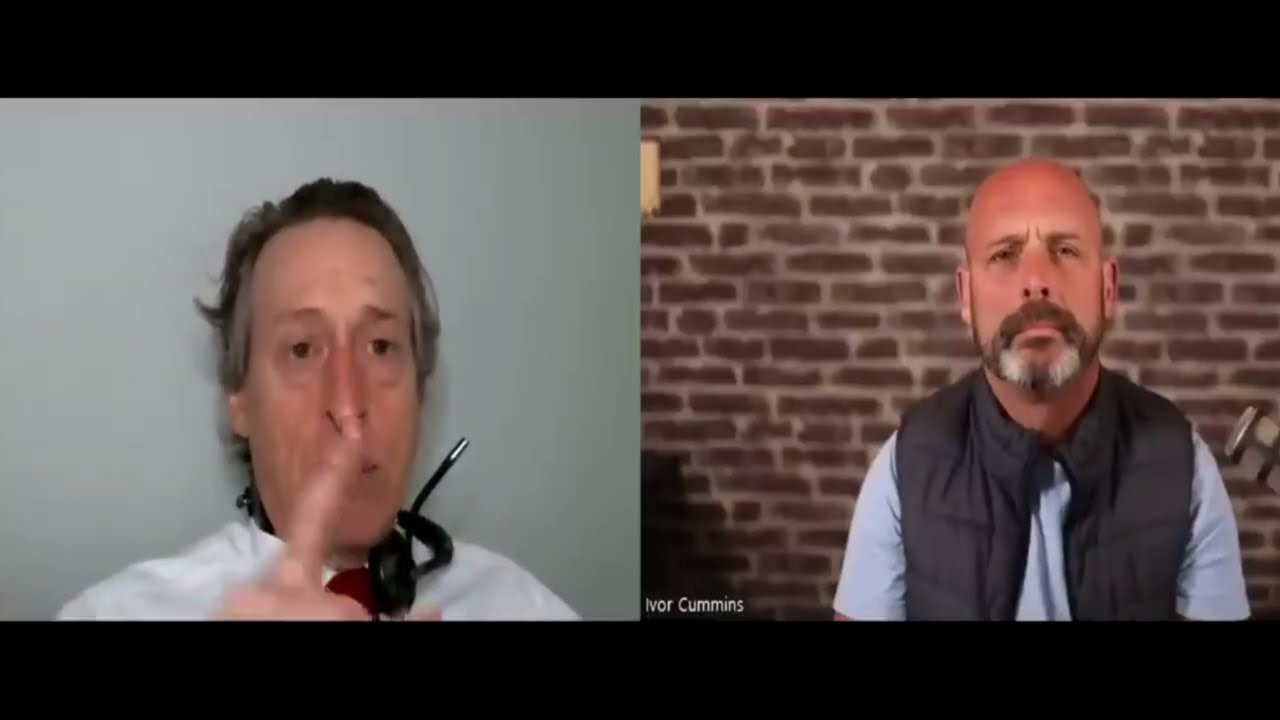This horizontal rectangular image depicts a split-screen view typical of an online video call, such as on Zoom. The left side shows an older man with short, wavy hair that is graying. He is in the process of speaking, with his right hand raised and one finger pointing up, adding emphasis. He is wearing a headset around his neck, resting on his shoulders, and his background consists of a plain gray wall.

On the right side, there is another man who appears to be engaged in the conversation. He is bald on top but has a brown beard with patches of white. He's wearing a puffy black vest over a short-sleeved t-shirt. His background is a brown brick wall. The name "Ivor Cummings" is displayed in white text at the bottom left corner of this square. The image captures a moment of interaction between the two individuals in a virtual meeting. The colors in the image include the peach tones of their skin, gray and brown shades of their hair and beards, and various tones from their clothing and backgrounds, creating a realistic depiction of an online conversation.